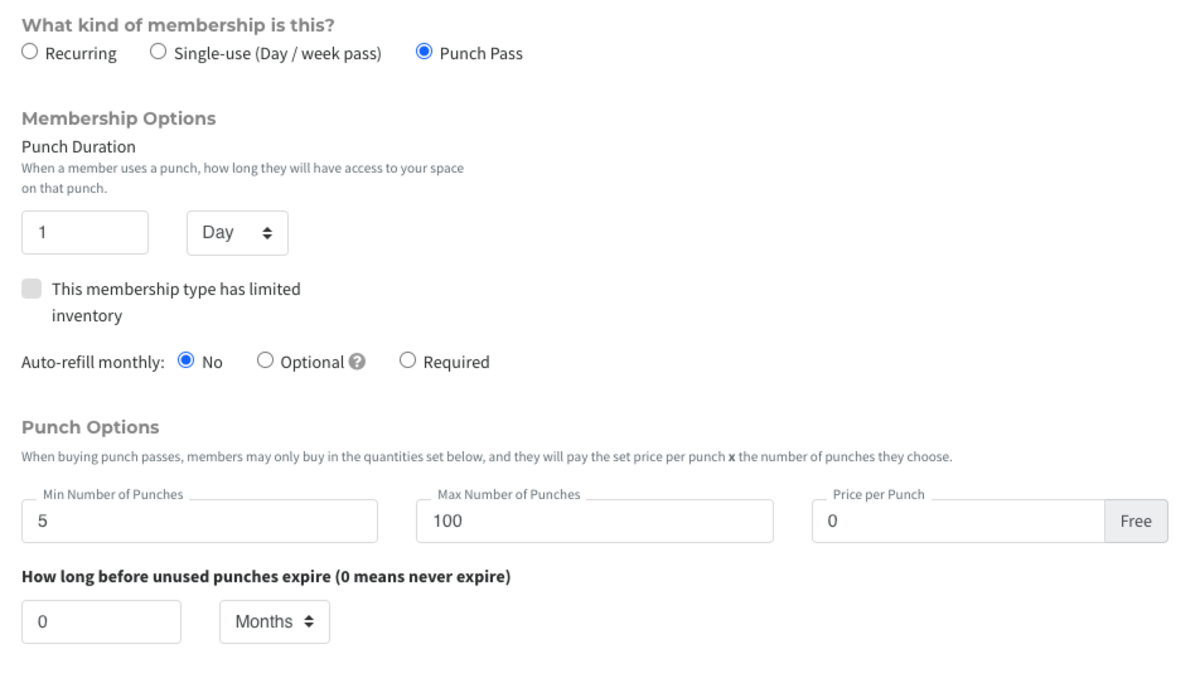The image features a clean, white background. At the top left corner, there's a label indicating the type of membership. Next to this, various membership options are presented in a horizontal row, each accompanied by an unfilled circle except for the 'Punch Pass' option, which is highlighted with a filled blue circle. The options from left to right read: Recurring, Single Use, (Day/Week Pass), and Punch Pass.

Below this row, the text "Membership Options" appears. Underneath it, a section titled 'Punch Duration' explains that it determines the length of time a member can access the space using a punch. Below this explanation, there is a textbox containing the number '1' with a dropdown menu adjacent to it displaying the unit 'Day.'

A checkbox below this area reads "This membership type has limited inventory," which is currently unchecked. Further down, there’s an "Auto Refill Monthly" section with three choices: 'No,' 'Optional,' and 'Required.' The 'No' option is selected, indicated by a filled blue circle, while the other two options remain unselected with hollow circles.

At the bottom of the image, the text "Punch Option" appears, followed by "When buying punch passes," concluding the description of the membership options.